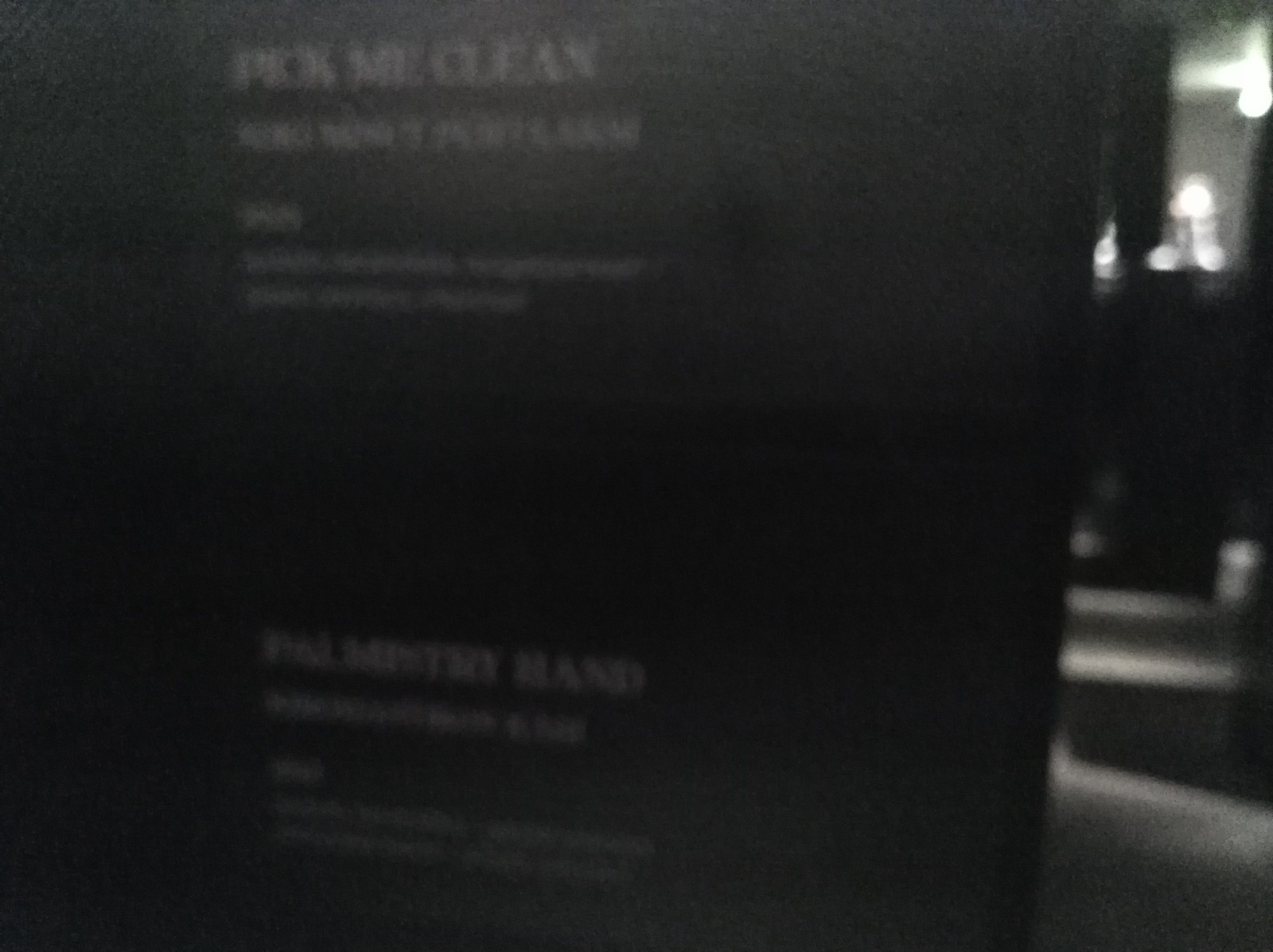In this blurry, rectangular black-and-white photograph, we see a dimly lit scene dominated by shadows and glowing lights. A prominent black sign with white text at the front of the image reads "Pick Mr. Clean" in capital letters, followed by a slightly blurred line and more text that appears to say "Pick Mystery Hand," though it is difficult to decipher. On the right side, the silhouette of a person, possibly seated at a desk, is partially visible, their arm close to their side. The image captures various light sources, including a bright display case in the corner and a glowing ceiling light, creating complex shadows on the floor. The graininess of the photo adds to its enigmatic atmosphere, with indistinct shapes that could be a garbage can, a box, or perhaps a small cup.